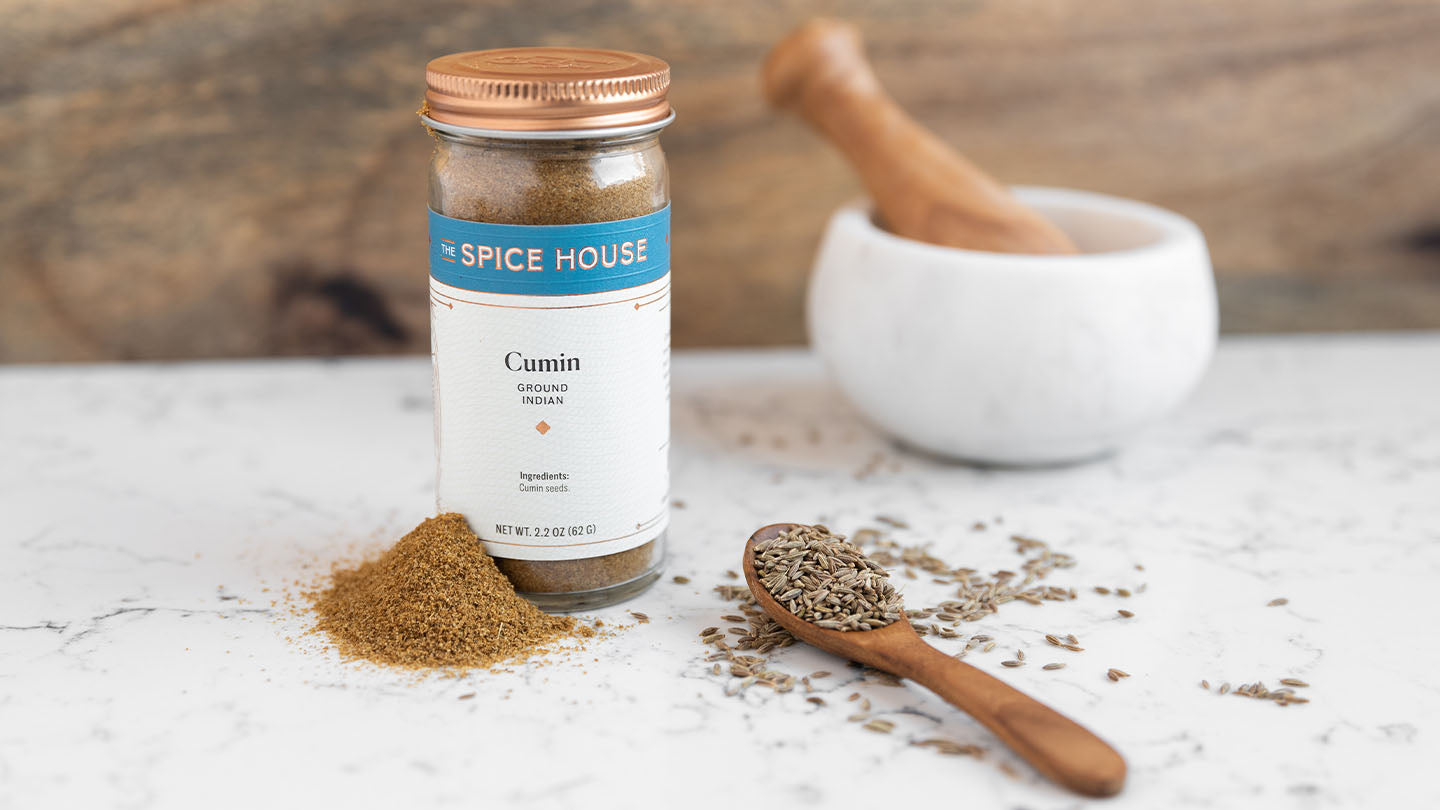In this stylized promotional photograph, the focus is a tall glass spice jar adorned with a coppery gold twist-off lid. The label on the jar, featuring a white background and a blue border at the top, prominently reads "The Spice House," followed by "Cumin, Ground Indian" and additional details including the ingredients and net weight of 2.2 ounces (62 grams). The jar visibly contains finely ground cumin. Positioned in the foreground is a small mound of the ground cumin next to a wooden spoon filled with whole cumin seeds, illustrating both the ground and seed forms of the spice. In the slightly blurred background, a white mortar and a wooden pestle can be seen, suggesting the process of grinding the seeds. The setting appears to be a white quartz countertop with light reflecting off the right side of the jar, enhancing its polished, promotional appeal.